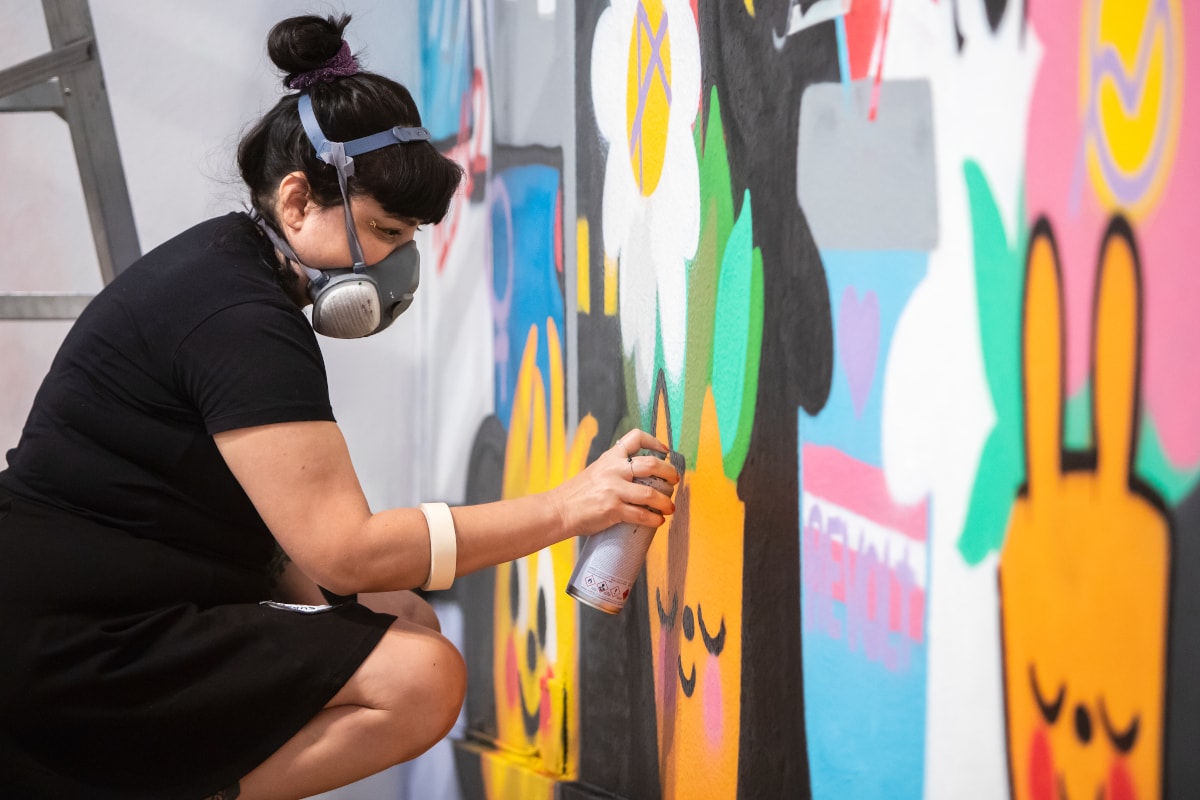In a photographic image captured in a horizontal landscape orientation, a woman is seen spray painting a colorful wall mural indoors. Positioned in the left third of the frame, she is crouching down with her knees and shins visible. The woman, who has her dark hair styled in a bun, is dressed in a short-sleeved black dress and a white bangle on her right wrist. She is using a spray paint can held in her right hand. A gray respirator mask covers her nose, mouth, and part of her chin, secured with straps, offering protection from the paint fumes.

The mural she is working on features various cartoon-style animal figures. The central section of her artwork includes an orange animal shape with black eyes and upside-down views, resembling a face with pointed ears. Adjacent to this, on the left, there's a similar figure with pointy ears, black eyes and mouth, and red cheeks, giving off a smiling expression. Further right, there is a gray sword-like object with what appears to be the letters "A-M-L-A-L" or "A-M-L-I-L-A-I" inscribed on its blade, although this text is slightly out of focus. Among the various hues and shapes, a light yellow animal can be seen with its eyes open and a joyful demeanor. The mural also includes splotches of blue, a white blob with an X on it, and a pink background adorned with a yellow check mark. Behind her, the wall features shades of gray, adding depth and contrast to the vibrant illustration she's creating.